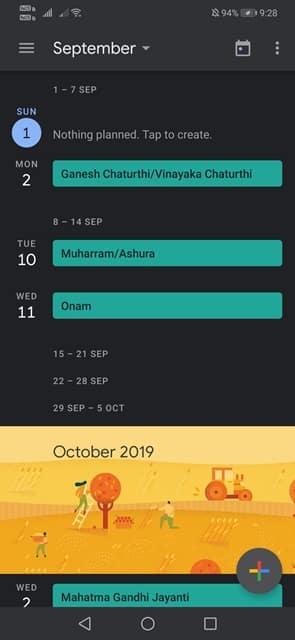Here is a detailed and cleaned-up caption for the screenshot described:

---

A screenshot of a calendar application with a black background. The calendar displays the month of September, and the year, indicated at the top as "October 2019." On the top left, there is a hamburger menu icon. Key dates and events are marked throughout the calendar:

- **1-7 September SCP:** A blue circular indicator marks this period, specifically highlighting Sunday, September 1st, labeled "SUN."
- **2 September:** This date is marked with a green rectangle and labeled as "Ganesh Chaturthi / Vinayaka Chaturthi," a Hindu festival.
- **8-14 September SCP:** Another highlighted week, though specific events aren't detailed in the initial description.
- **10 September:** This date is marked with a green rectangle, labeled "Muharram," signifying an Islamic event.
- **11 September:** Indicated with the label "ONM," though further details aren't given.
- **15-21 September SCP:** Another week marked without specific events detailed.
- **22-28 September SCP:** This week is highlighted similarly to previous ones.
- **29 September - 5 October:** The end of September is marked, transitioning into October.

In the bottom right corner, there is a grey circle with a plus sign in the middle, surrounded by the colors of the Google logo, suggesting an option to add new events.

---

This cleaned-up version preserves all provided details while organizing them clearly and cohesively.